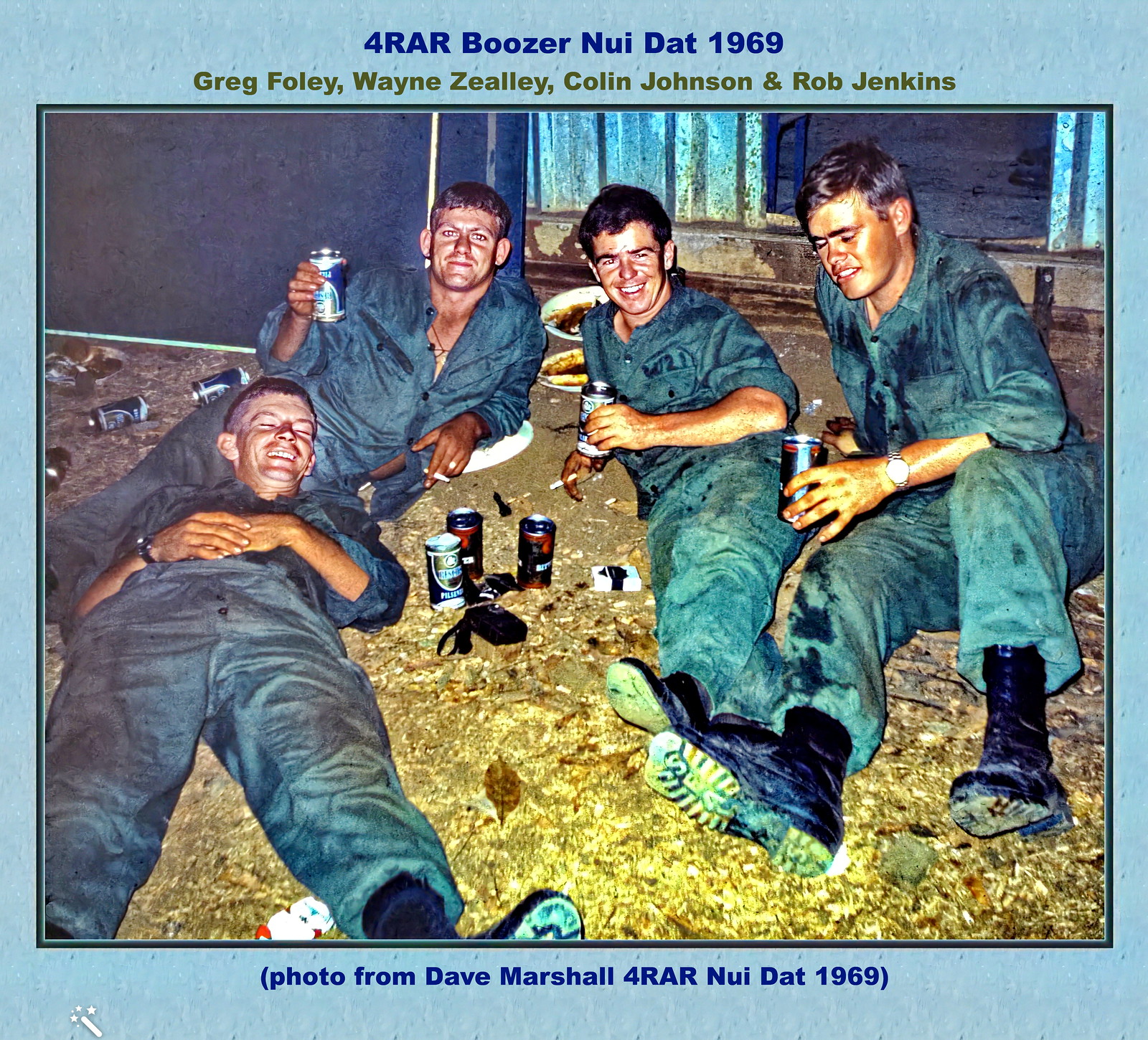The image depicts a relaxed moment among four young men, likely military personnel, lounging on a dirt floor covered with leaves and debris inside what appears to be a barn or shed. At the top of the photograph, the text reads, "For R.A.R. Buzier, Nui Dat, 1969," followed by the names of the men: Greg Foley, Wayne Zealy, Colin Johnson, and Rob Jenkins. Below the photo, it notes, "Photo from Dave Marshall for R.A.R. Nui Dat, 1969." The men, dressed in dark gray or greenish-gray jumpsuits and combat boots, are seated or lying on the ground, each holding an aluminum can, presumably of beer, with more empty cans scattered around them. One man reclines with his head resting on another's knee while the other three are either posing or aware of the camera. Additional details include visible packs of cigarettes, plates with food, and possibly a camera in the background. Subtle touches like the blue border and the rustic setting underscore the casual camaraderie and setting of this 1969 snapshot.